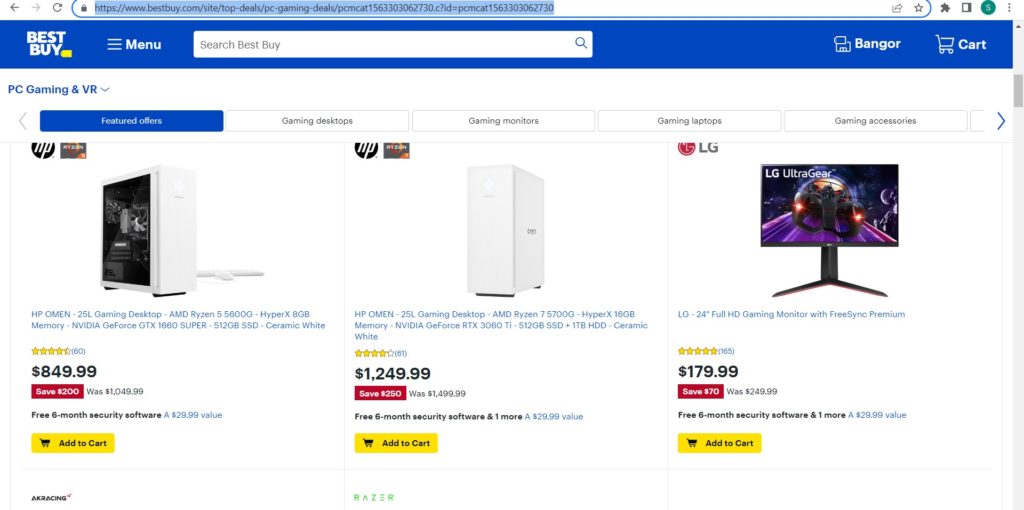This screenshot captures the interface of the Best Buy website displayed on a Mac computer, as evidenced by the layout distinctive to macOS. 

At the top, the navigation bar is visible with a highlighted URL in blue, indicating it is currently selected. The left side of this bar features a back arrow, while the right side showcases several system icons. 

Below the navigation bar, the website's header banner appears prominently. On the left side, the Best Buy logo is displayed in white against a blue background. To the right of the logo is a "Menu" icon represented by three horizontal lines. Further along is a white search bar, followed by icons labeled "banger" and "cart."

The section immediately below the header is set against a white background and centers around "PC Gaming and VR." This section is organized with five navigational options, flanked by left and right arrows for scrolling. The active option is highlighted in blue, indicating the current page.

The main content area features three product columns. The first two products are from HP, and the third is from LG. Each product listing includes a logo, detailed information, and pricing. A red button is below each product listing, likely for additional actions such as viewing details. Beneath these, a yellow "Add to Cart" button, with black text, is prominent.

Finally, the very bottom of the page contains a small section of text in blue, too tiny to be legible from the screenshot.